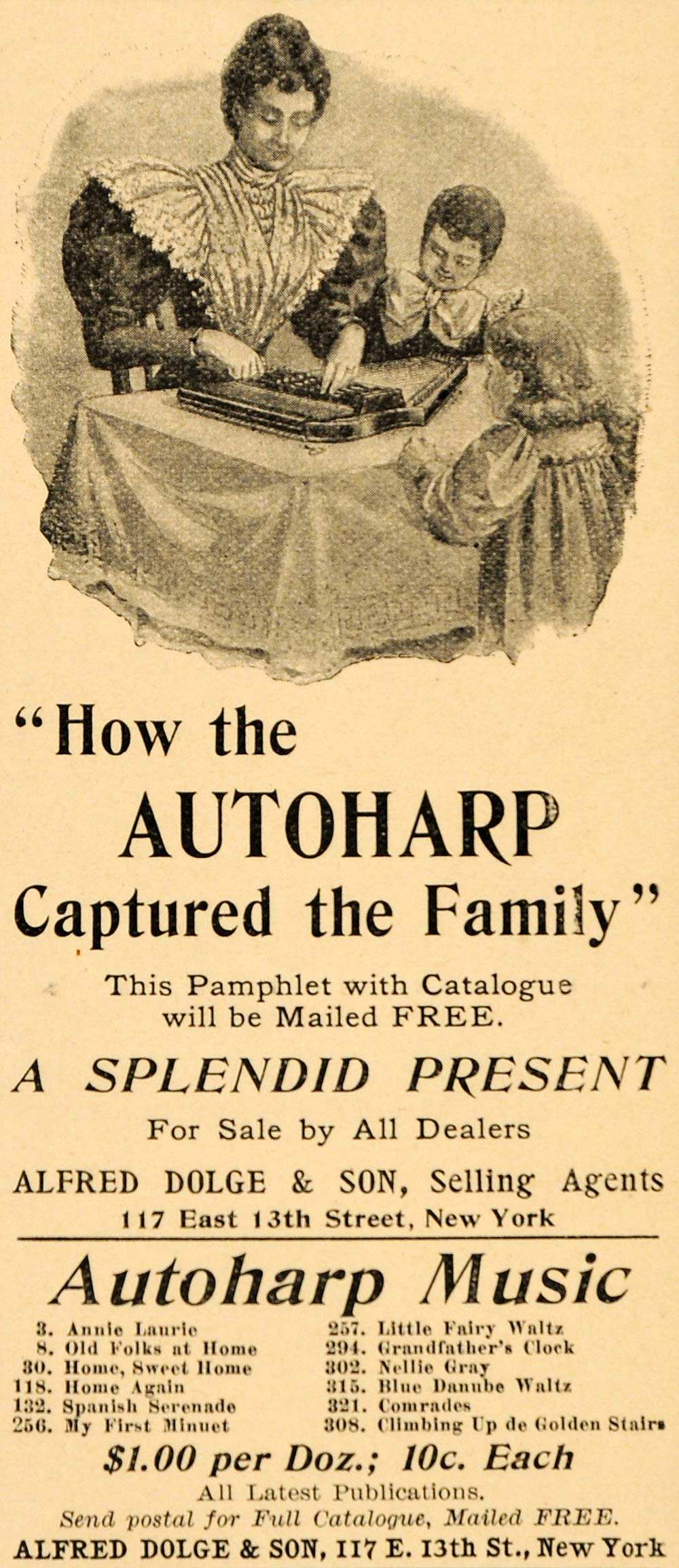This image showcases a vintage newspaper advertisement, likely from 50 to 60 years ago, featuring a mother and her two children dressed in ornate Victorian-era clothing. The mother, with her dark hair styled in a bun, is wearing a frilly dress with a white collar. One child, a boy, stands beside her, adorned with a large white bow on his shirt, while a little girl with hair in ringlets stands at the opposite side of the table facing the mother. At the center of their attention is an auto harp on a table covered with a linen cloth. The caption beneath the drawing reads, "How the Auto Harp Captured the Family." The advertisement also announces the availability of a free pamphlet and catalog, declaring it a splendid present, available through all dealers. Selling agents Alfred Dolgen and Son are mentioned at their address, 117 East 13th Street, New York. Additionally, the ad states that Auto Harp Music is priced at $1 per dozen or 10 cents each, with all the latest publications being sent by postal for the full free catalog.